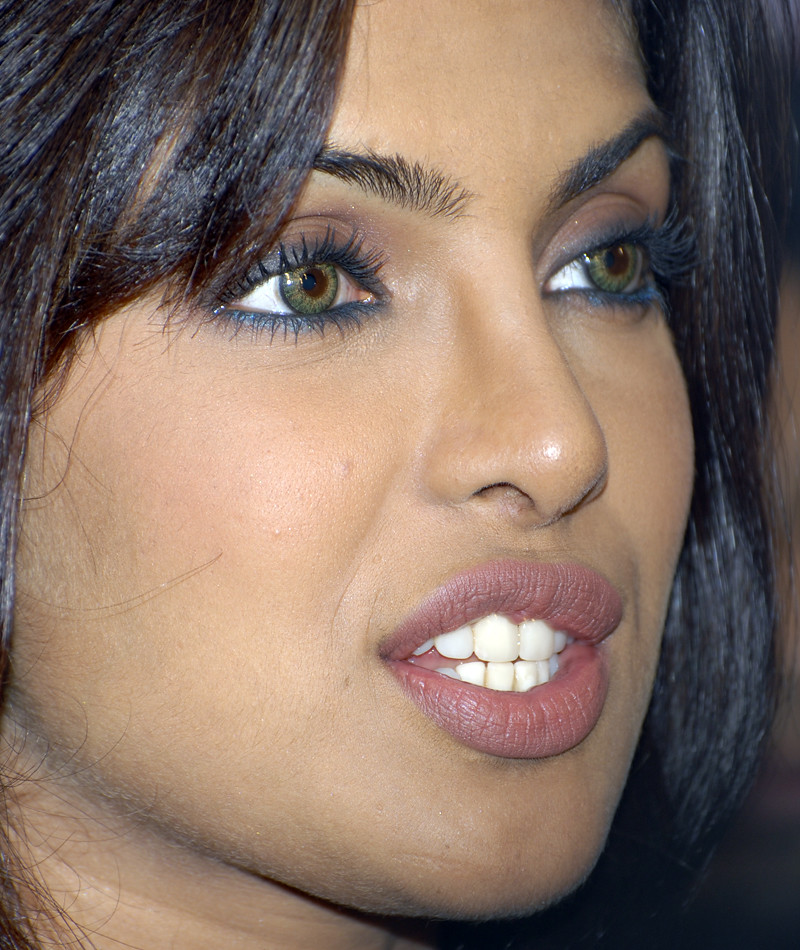This is a close-up color photograph in portrait orientation capturing a young woman in her late 20s to early 30s. She has black, slightly longer than shoulder-length hair and dark eyebrows. Her green eyes, adorned with blue eyeliner, are looking slightly towards something off-camera to the right. Her lips, partially parted to reveal both rows of white teeth, are accentuated with red lipstick. The image focuses intently on her face, which has pale golden skin. Despite some varying descriptions, it appears that she might be talking. The backdrop behind her is blurred due to the focused lighting on her face, contributing to the photograph's realism and representational style.